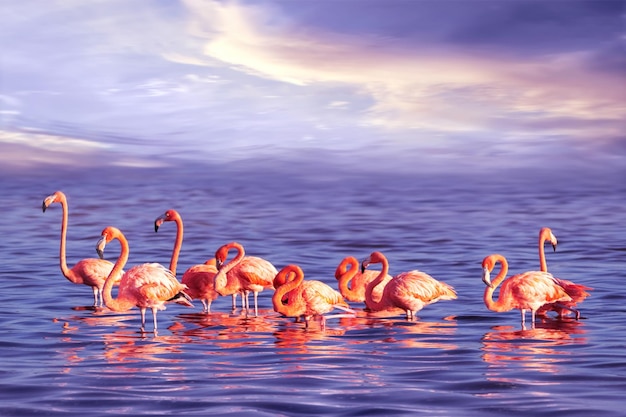The photograph captures a serene scene of a pastel-colored ocean, blending hues of purples and pinks, where a group of nine flamingos wade in the tranquil water. The flamingos display a vibrant spectrum of pinks and corals, with some standing tall on their long necks while others are gracefully crouched, their heads arched and beaks nestled into their breasts in a preening pose. The horizon seamlessly merges with the water, creating an almost indistinguishable line as the same soft shades of light purple and violet ascend into the sky. Wispy, white clouds scatter across the ethereal backdrop, adding texture to the tranquil scene. The reflections of the flamingos ripple gently in the water, accentuating the calm and dreamlike quality of the image.